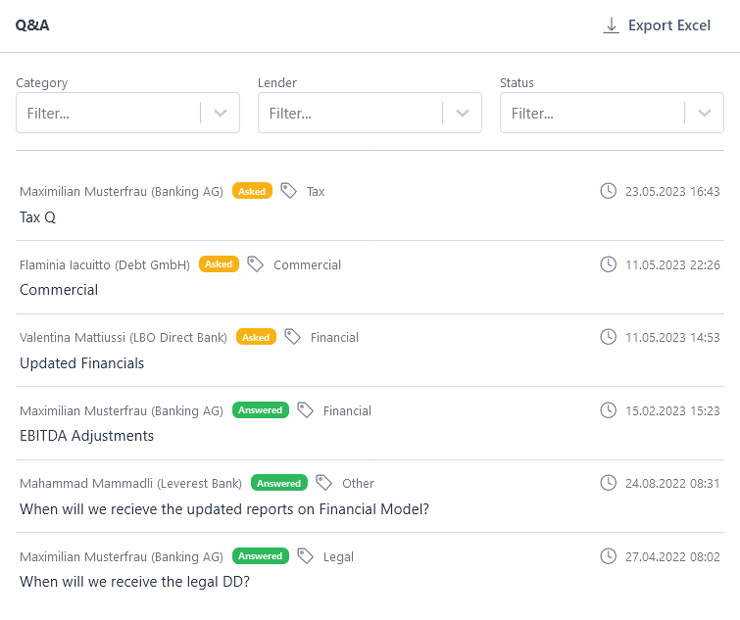The image is a screenshot of a computer screen displaying financial banking information. In the top left corner, there is a bold "Q&A" label. On the top right, a download icon with an arrow pointing downwards is labeled "Export Excel" in bold text. Below these, there's a row with three filter headings: "Category" on the left, "Lender" in the middle, and "Status" on the right. Each of these headings has a corresponding drop-down menu with the default word "Filter".

Beneath these filters is a table containing rows of financial information that appear to be questions and answers related to banking. Each row includes the name of the person who asked the question, the associated bank (e.g., tax, commercial, or financial), and the date and time the question was asked or answered. Questions that have been asked are highlighted with a yellow circle, while answered questions are marked with a green circle.